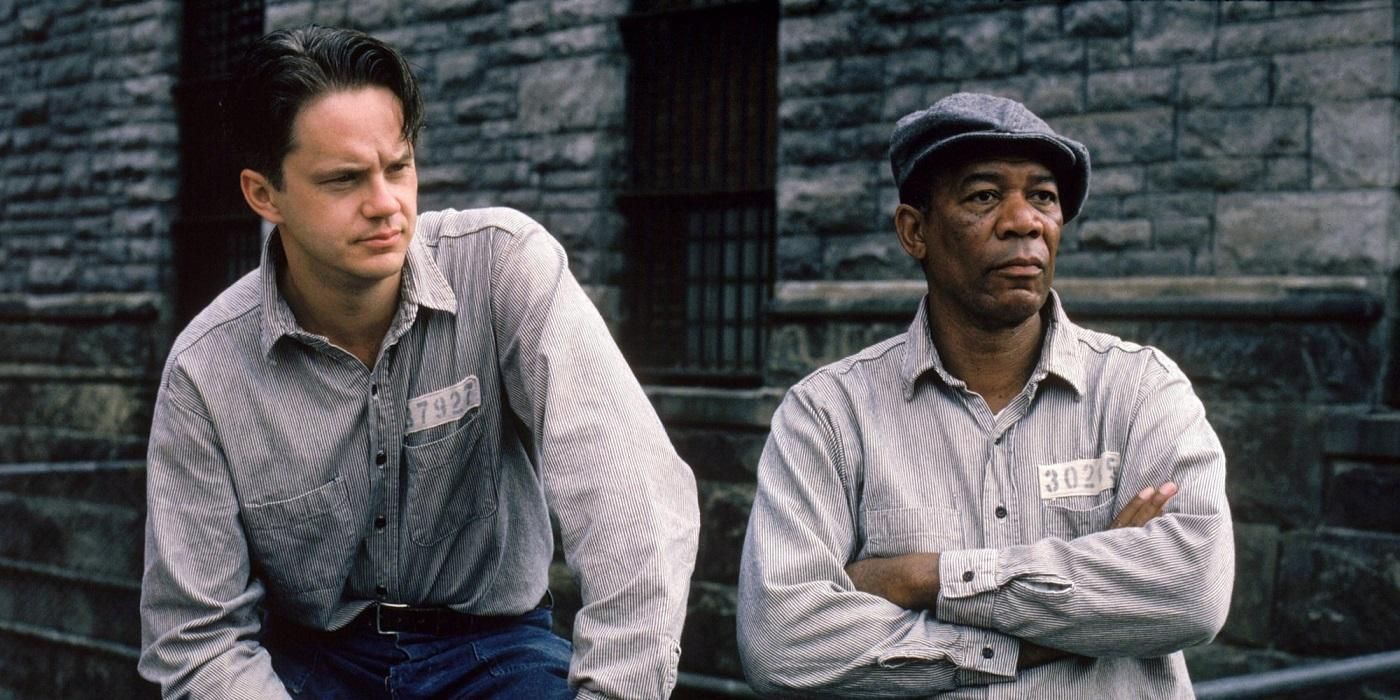This is a detailed color still from the 1990s movie "The Shawshank Redemption," based on a book. The scene features two prison inmates against a backdrop of a substantial grey brick wall with metal black grates. The inmate on the left, portrayed by Tim Robbins, has dark, slicked-back hair and a stern, frowning expression with pinched brows. He is wearing a grey button-up, long-sleeved shirt with the inmate number "7927" above the left chest pocket, paired with a black belt with a silver buckle and blue jeans. On the right is actor Morgan Freeman, wearing a grey beret and a matching grey prison shirt with the number "30285" visible. His arms are folded as he stands next to Robbins. Both actors are positioned against the sturdy, imposing backdrop that further highlights the harsh environment of their incarceration.